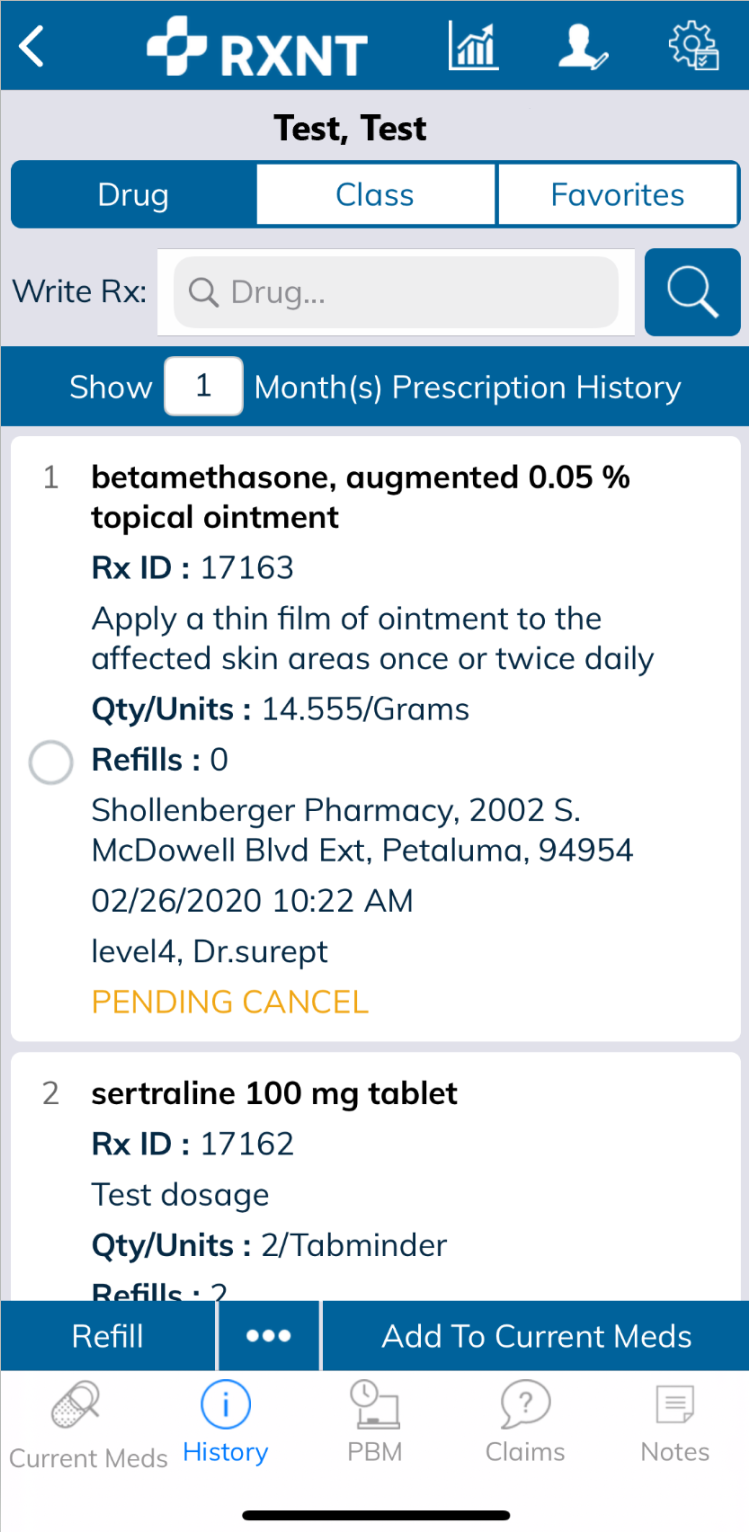**Detailed Description of the Image:**

The image is a screenshot of a mobile interface from an online pharmacy platform, designed specifically for a mobile device. At the very top of the screenshot, there is a blue navigation bar featuring the letters "R", "X", and "T" in white text. Adjacent to this, there is an icon consisting of four white squares surrounding a central blue square. 

Below the navigation bar, there are several icons: 
1. A chart icon.
2. An icon depicting a patient.
3. An icon resembling a lock symbol.

Directly underneath this, in black text, the screenshot displays "test, test." Below this text, there are three buttons: "Drug", "Class", and "Favorites." The "Drug" button is highlighted in blue, while the other two are in white. Underneath these buttons, there is a field labeled "Write RX" followed by "Drug..." and a search bar button.

The screenshot then shows a section detailing a patient's prescription history for one month. The specific medication listed is "bethamethasone augmented 0.05% topical ointment" with the prescription ID (RxID) of 17163. The instructions indicate: "Apply a thin film of ointment to the affected skin areas once or twice daily." The quantity prescribed is 14.555 grams, with zero refills available. 

The prescribing pharmacy is Schallenberger Pharmacy, located at 2002 Aspect Owl Boulevard, Extension Petaluma, 94954. The prescription date is February 26, 2020, and the time noted is 10:22 a.m.